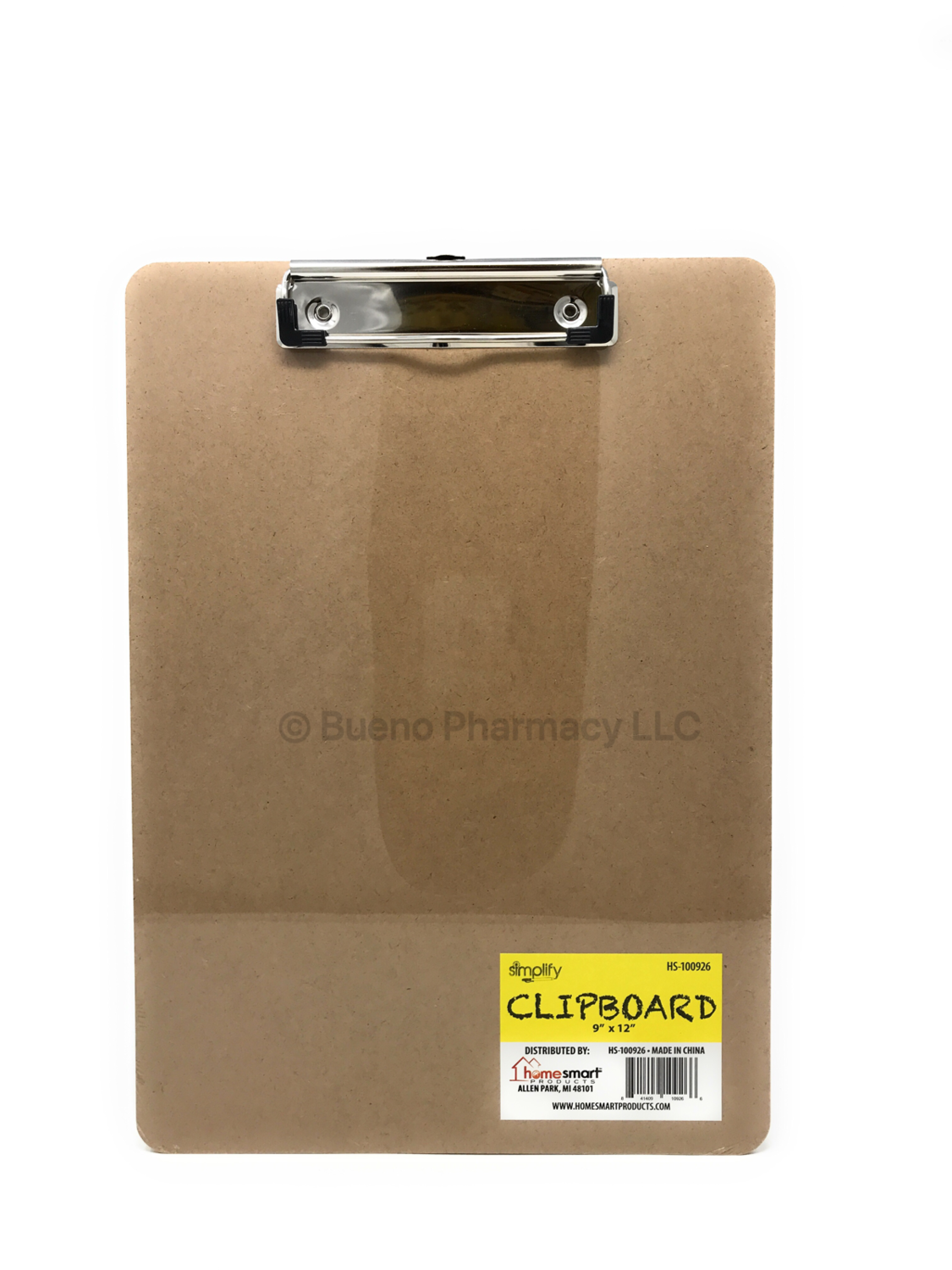This image is a vertical, cropped photograph of a brown wooden clipboard with a metal clip, set against a plain white background, likely intended for online sale. The silver clip at the top is affixed with two screws, creating a slight shadow that might appear as a stain. Prominently displayed in the center of the clipboard is the label reading "copyright Bueno Pharmacy LLC." The clipboard appears new, suggested by the intact barcode label in the lower right-hand corner. The label's upper section is yellow, featuring the text "Simplify Clipboard 9x12" in black, while the bottom section is white, displaying the barcode and manufacturing details, including "HS100796" and "Made in China." The brand name "HomeSmart" is highlighted in red and black text on the label, indicating the clipboard's likely branding.